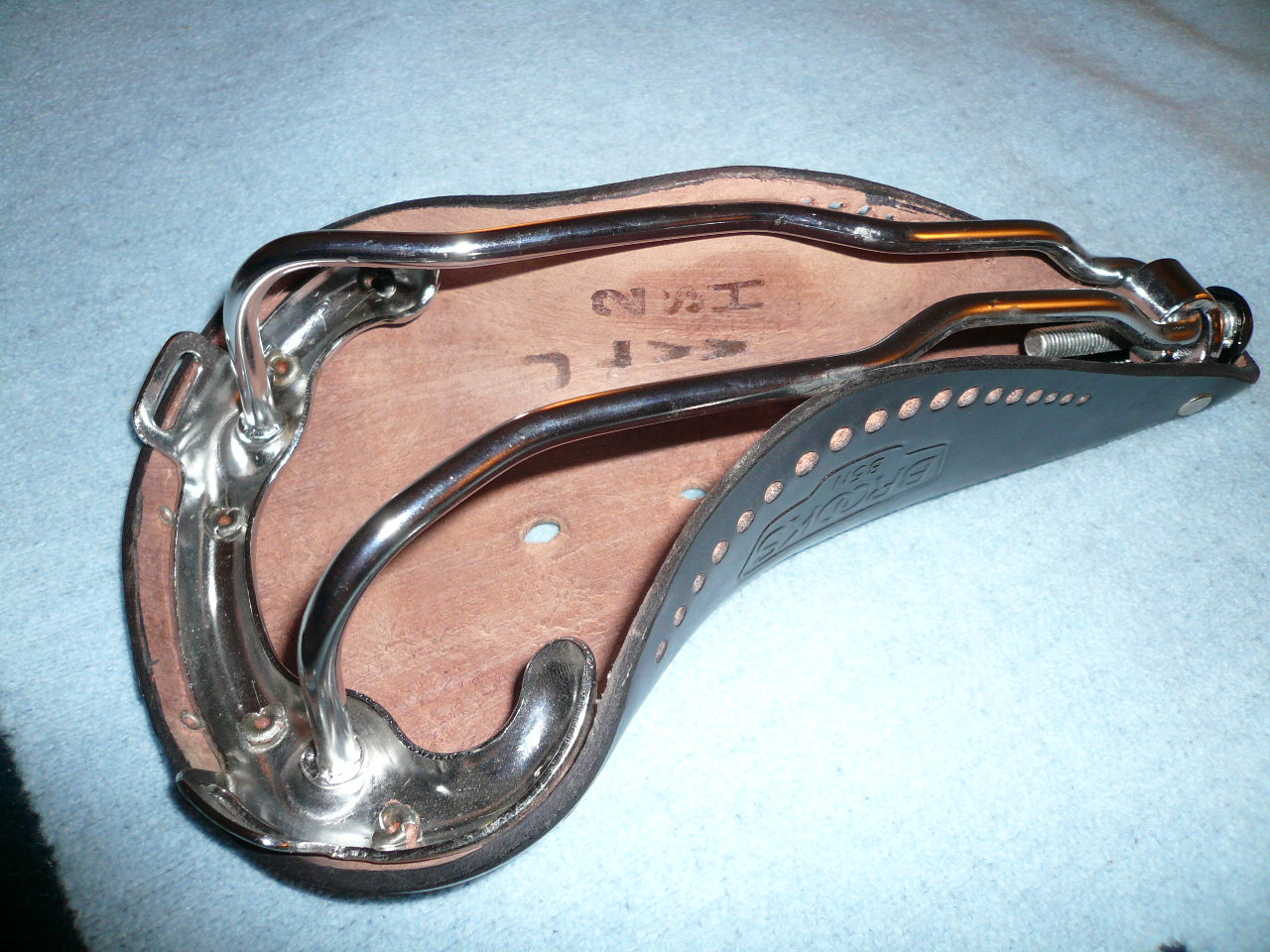The photograph shows a detailed view of a dark brown (almost black) leather bicycle seat resting upside down on a light blue fabric surface. The seat is crafted from thick leather that wraps around a wishbone-shaped stainless steel frame, which is welded to a C-shaped metal piece for support and structure. This distinctive outline, resembling a seashell with turned-up ends, features holes punched along the sides and an embossed text, though the text is illegible. A silver metal component spans the back and extends downward, suggesting a clip mechanism, adding to the complexity of the design. The item is positioned centrally on a light blue cloth or towel that covers a table, providing a contrasting background that highlights the intricate details and textures of the seat.